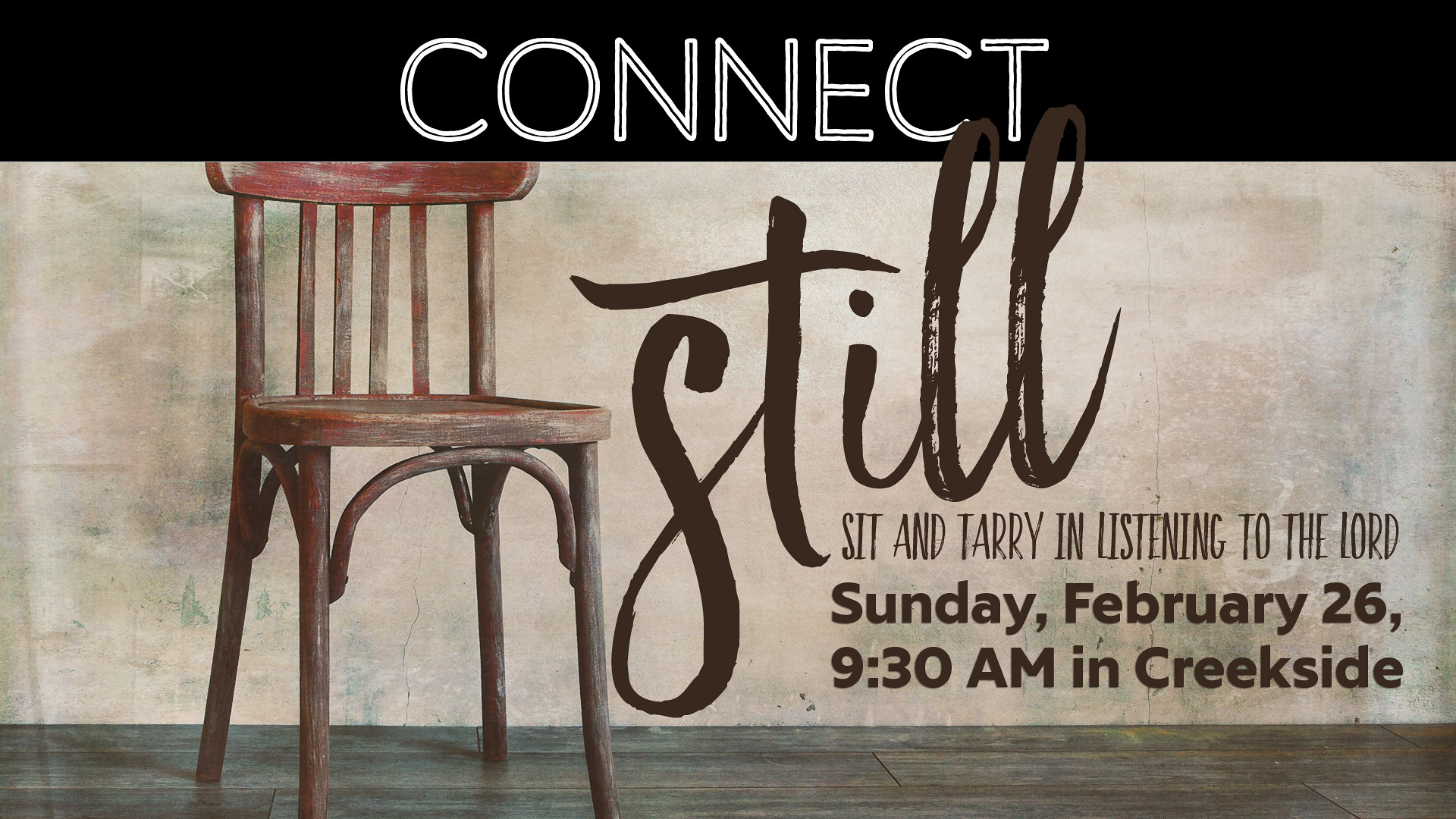The image serves as an advertisement for a religious gathering, featuring an old-fashioned, weathered wooden chair positioned against a beige wall with a brown floor, suggesting an indoor setting. At the top of the advertisement, a black bar with white text prominently displays the word "CONNECT." To the right of the chair, the word "STILL" appears in cursive script. Beneath it, the phrase "Sit and tarry in listening to the Lord" is written in dark brown text. The advertisement details the event will be held on Sunday, February 26th at 9:30 a.m. in Creekside.